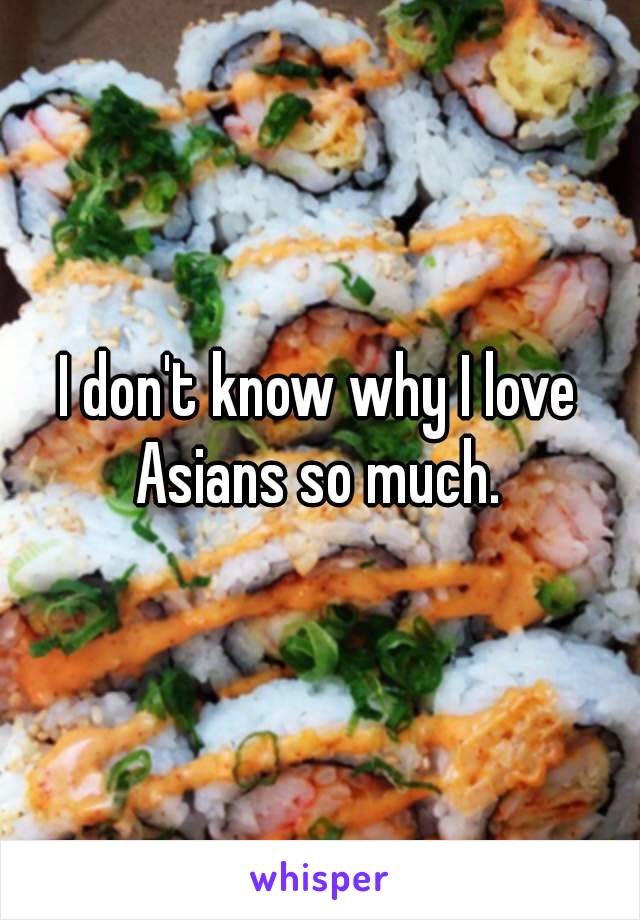This close-up image features four rows of cut sushi rolls, commonly resembling a California roll, each wrapped in seaweed with white rice on the outside. Inside, the rolls appear to contain crab and something pinkish, while the tops are adorned with a spicy mayonnaise drizzle, chopped scallions, and sesame seeds. The sushi is the sole focus of the image, with no visible background. Superimposed over the sushi in bold white lettering outlined in black, the text reads, "I don't know why I love Asians so much." Additionally, at the bottom of the image, a white banner contains the word "Whisper" in purple letters.